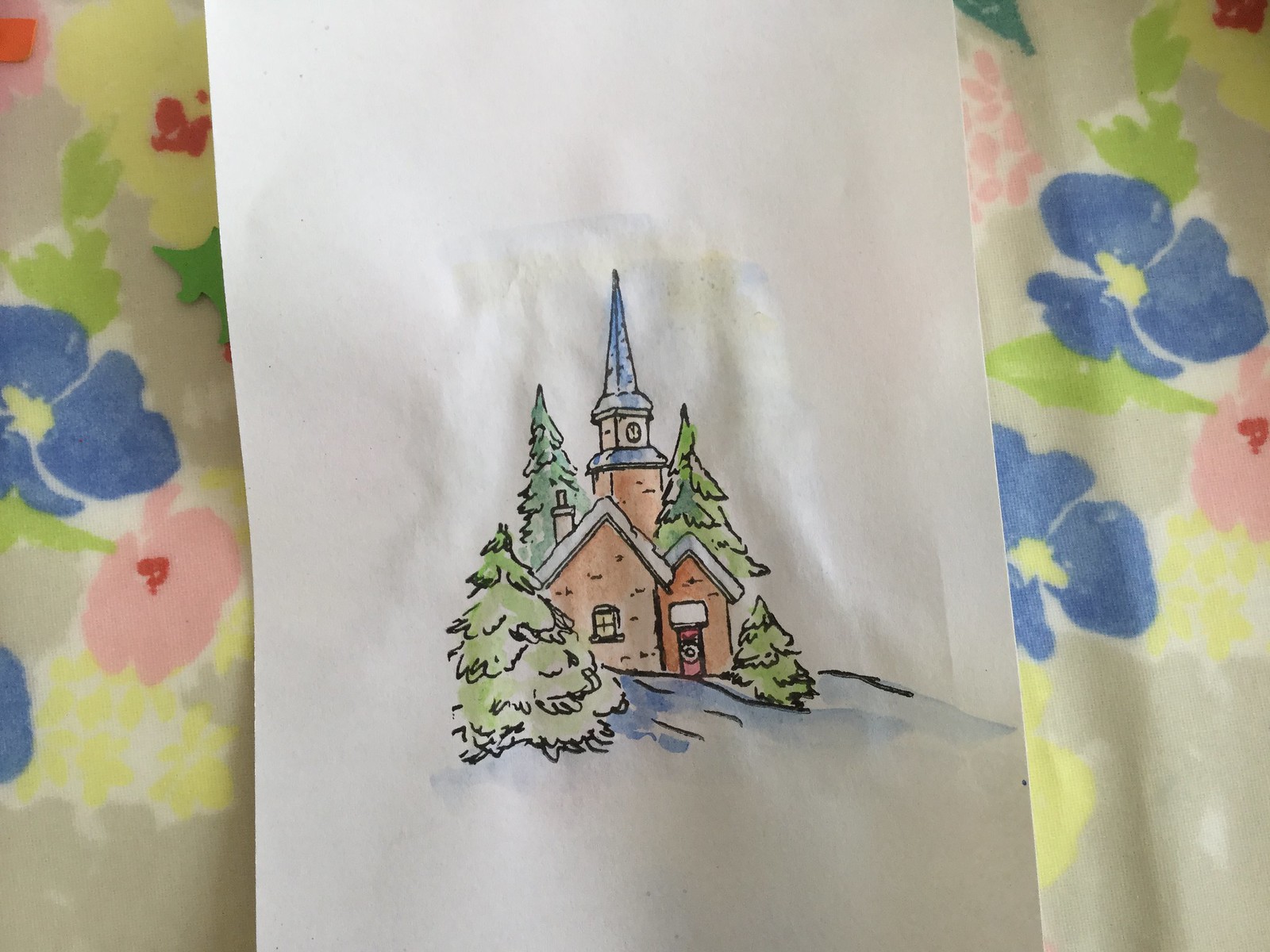In this captivating watercolor painting, a serene church with a light brown facade and a striking clock tower adorned with a blue steeple takes center stage. The church is encircled by four towering evergreen trees, two of which nearly reach the height of the clock tower. A bright red door marks the entrance of the church, adding a vivid contrast to the wintry scene, as hints of snow blanket the ground in front. The painting rests on an elegant gray and white cloth, intricately patterned with delicate blue, yellow, and pink flowers, providing a charming backdrop that enhances the overall aesthetic of this tranquil artwork.